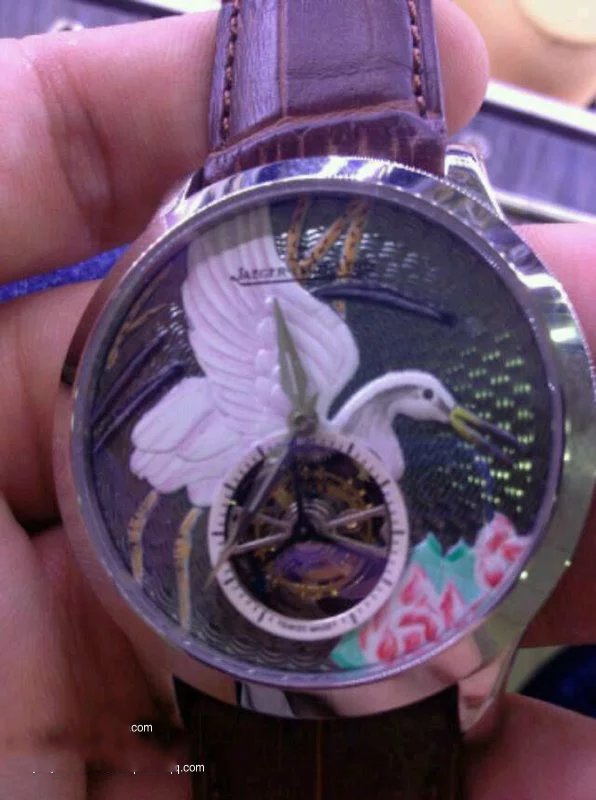This image showcases an elegant women’s watch with a distinctive purple alligator leather band. The watch features a round face adorned with intricate details. At the center of the watch face, there is a bird that resembles a dove, though its unusually long beak suggests it may be a different species. The bird, which has long legs, stands amidst delicate pink flowers positioned at the bottom of the watch face. The timepiece is devoid of numerals, making it necessary to approximate the time using the silver hands, which blend subtly into the intricate design. The watch is held gracefully by what is likely a woman's hand, emphasizing its feminine appeal. The bottom of the image contains text that includes "com," possibly part of a web address or brand name.